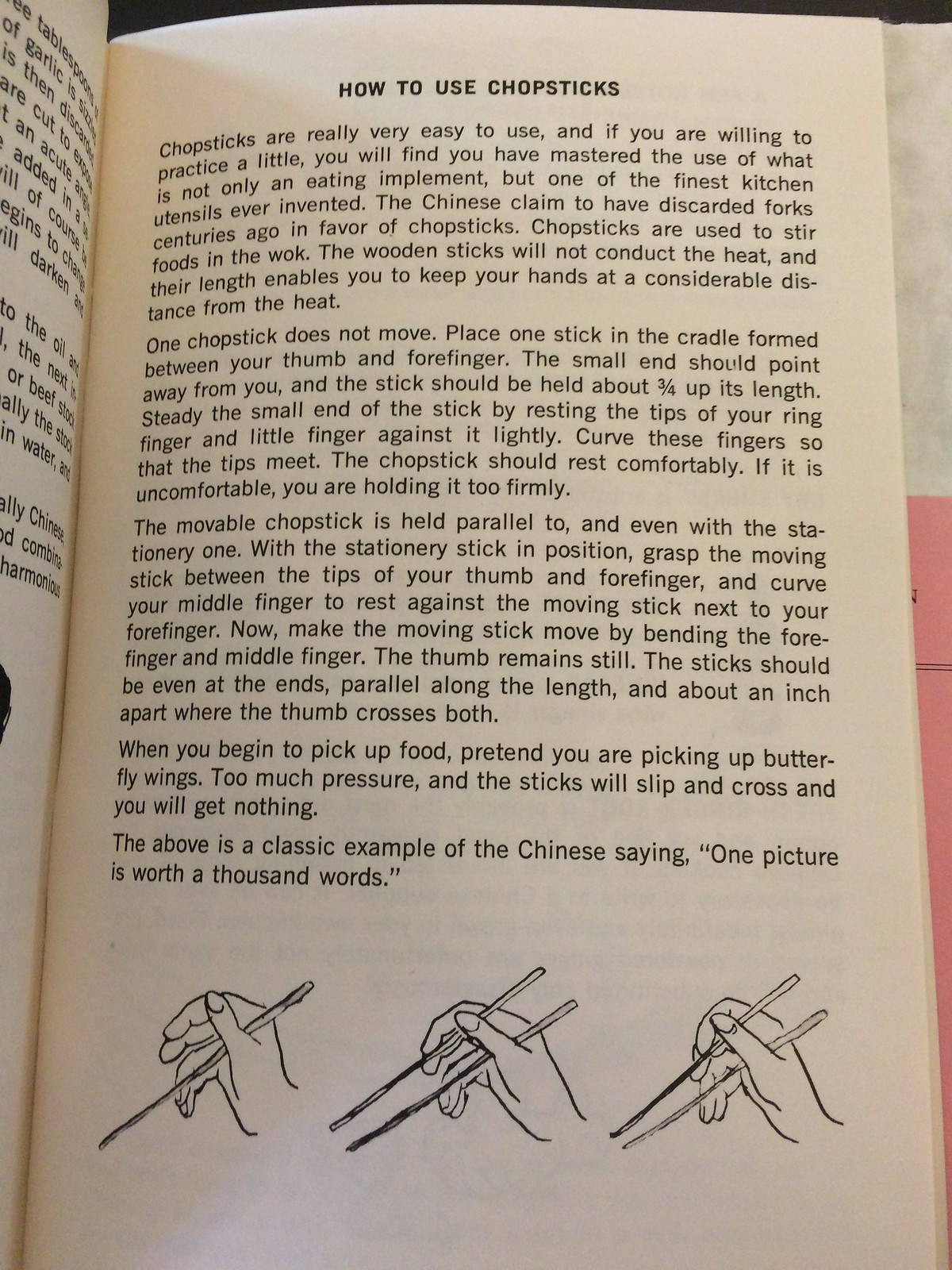The photograph captures an excerpt from a book, prominently featuring a page titled "How to Use Chopsticks." The right page is fully visible, while the left is partially obstructed, showing incomplete text. The page provides a comprehensive guide on the use of chopsticks, emphasizing their ease of use and effectiveness with practice. It details their dual role as both an eating implement and a cooking tool, highlighting their use in stirring foods in a wok without conducting heat. The page is adorned with three black-and-white illustrations at the bottom, resembling pencil or pen drawings, that sequentially demonstrate the proper technique for holding and using chopsticks. The first image shows a hand holding one chopstick, the second depicts the hand holding two chopsticks, and the third illustration demonstrates the chopsticks in action, pinching together as if to pick up food. The text advises holding one chopstick stationary and using the other to move, with detailed steps on finger placement and movement to master the technique. It concludes with a quote, "One picture is worth a thousand words," underlining the instructional value of the illustrations.